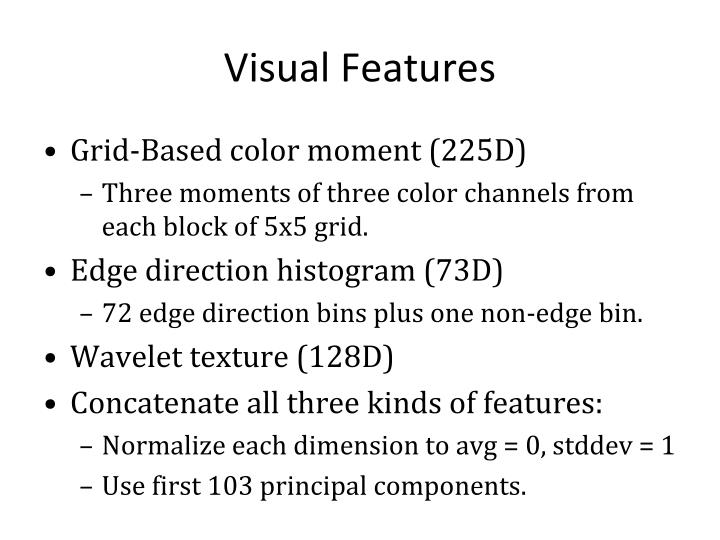The image is a slide with a white background and black text, resembling a PowerPoint presentation. The centered heading at the top reads "Visual Features." Below it are four left-aligned bullet points detailing various visual features. 

1. The first bullet point states "Grid-Based Color Moments (225D)" with a sub-bullet explaining "Three moments of three color channels from each block of a 5x5 grid."
2. The second bullet point is "Edge Direction Histogram (73D)" followed by a sub-bullet that elaborates "72 edge direction bins plus one non-edge bin."
3. The third bullet point is "Wavelet Texture (128D)."
4. The fourth bullet point instructs to "Concatenate all three kinds of features:" followed by two sub-bullets. The first specifies "Normalize each dimension to AVG = 0, STD DEV = 1," and the second advises to "Use first 103 principal components."

The text is detailed and precise, intended to convey technical aspects of visual feature analysis.